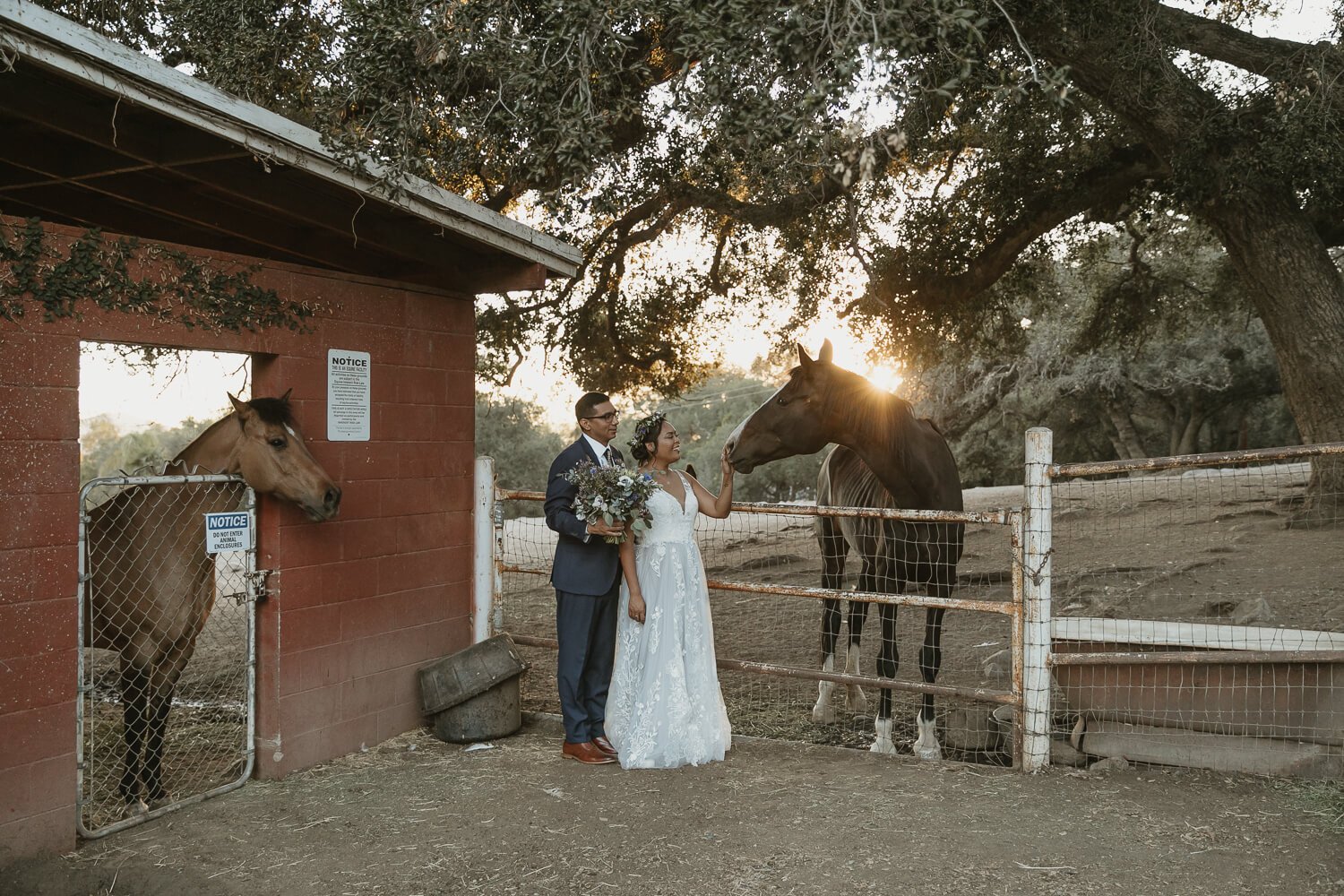In this detailed wedding portrait set in a horse farm, a bride and groom stand prominently. The bride wears a sleeveless, traditional white wedding gown with a dip neckline and flowers adorning her hair, while the groom is in a navy blue suit with a white shirt and brown shoes, holding the bride's bouquet. The groom has short black hair and wears glasses. Both are of African descent and are lovingly engaging with a horse behind a gated rail fence, with the bride touching its nose. Behind them, a red brick building with a "Notice: Do Not Enter Animal Enclosures" sign frames the scene, and another horse pokes its head outside a nearby wired iron gate. Additional farm elements such as baskets and utensils for feeding are visible, along with large trees, rocks, hills, and bright sunshine that complete the rustic and romantic setting.